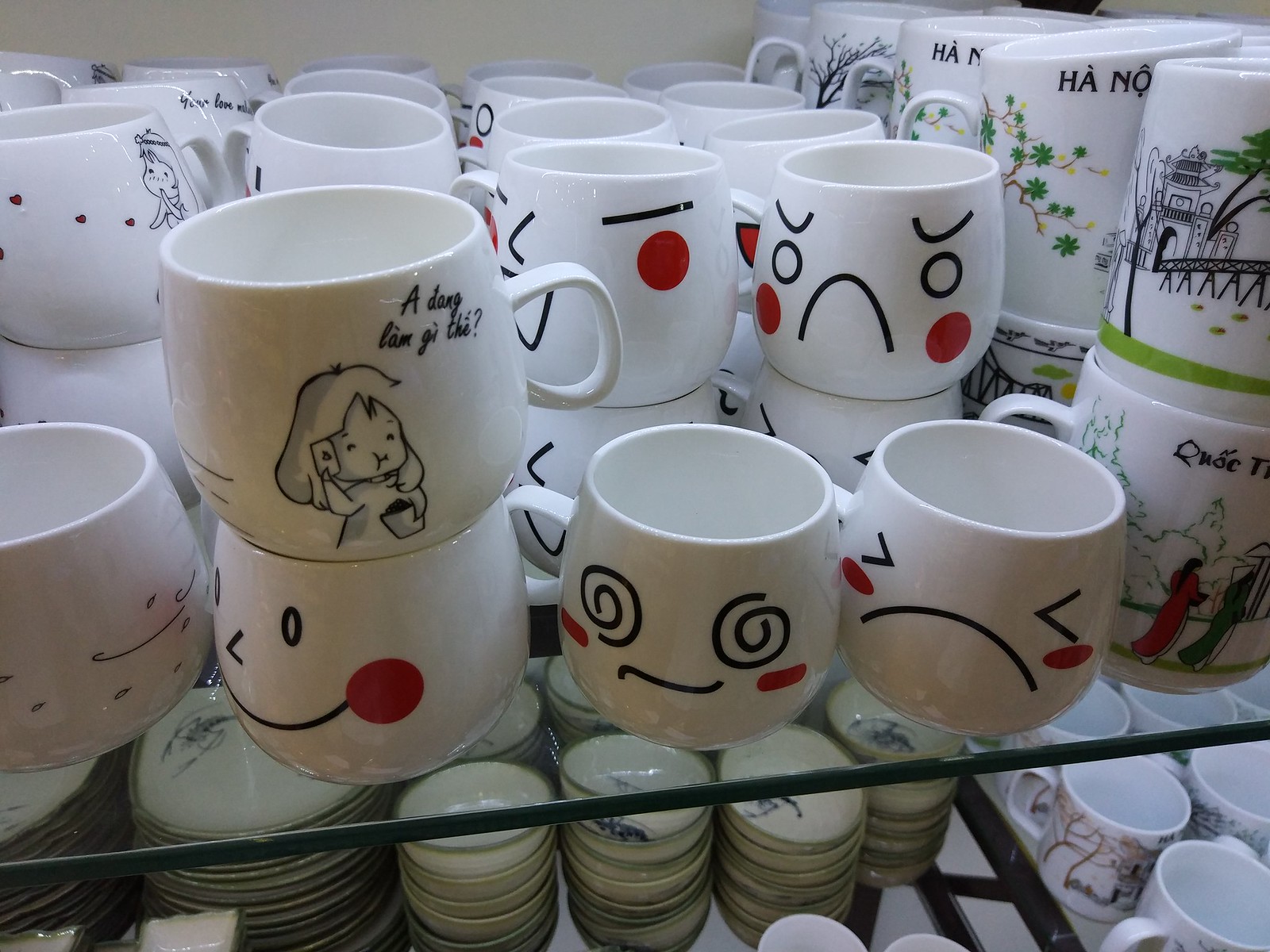This detailed photograph captures an array of intricately designed mugs displayed on a glass shelving unit, likely in an Asian-influenced store. The top shelf showcases an assortment of white mugs, some stacked two high. Each mug features a variety of simple, expressive faces rendered in black lines with red accents. The faces range from happy and laughing to sad and confused, each expression distinct yet cohesive in their minimalistic style. Among these mugs, one stands out with a black-and-white sketch of an anime-style girl, who is depicted holding a phone to her ear and perhaps a cup of food. The mug is adorned with Vietnamese text that reads, "Đông làm gì thế?" 

In the lower right corner, another row of distinctively styled mugs is visible, characterized by more ornate Asian artwork in green, black, red, and brown lines, which contrasts with the simplicity of the emoji faces. Below this shelf, there is another level of storage featuring a variety of ceramic mugs and small plates, likely intended for soy sauce or other condiments. This carefully composed image emphasizes the diverse artistic expressions and cultural influences embodied in the mug designs.